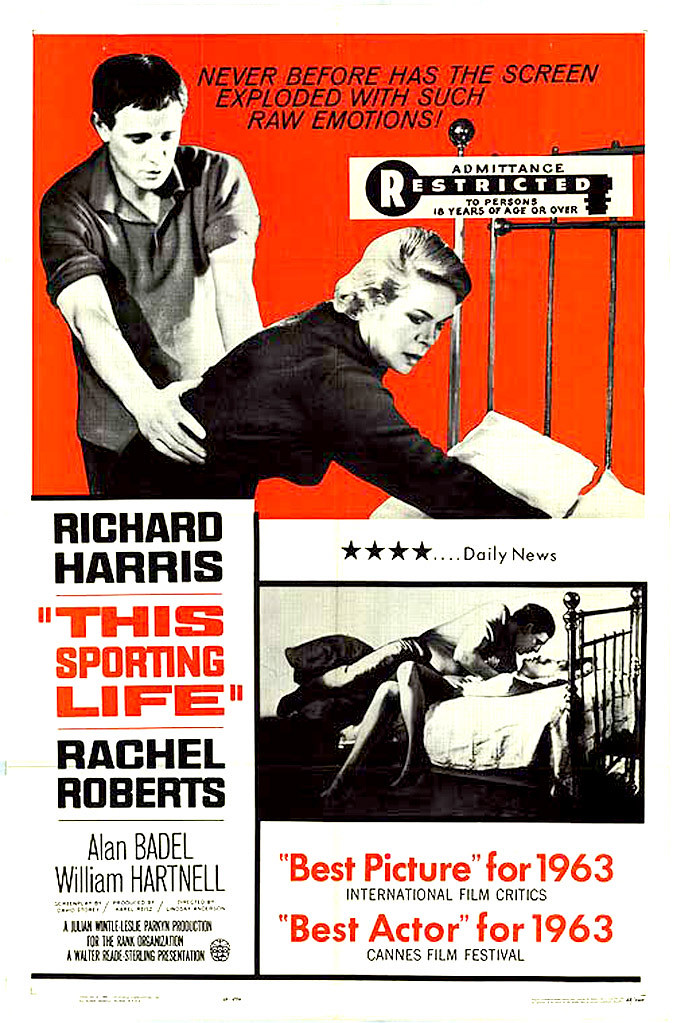The image is an advertisement for a movie restricted to viewers 16 years and older. The poster features a bright orange-red background in its top half, where a larger image depicts a man embracing a woman who is bent over, with the text, "Never before has the screen exploded with such raw emotions." Below this, two smaller thumbnail images are positioned side by side: one showing a man atop a woman in a bed, evoking a seductive scene typical of the 1960s. The text is a mix of red and black print, with accolades including "Best Picture for 1963, International Film Critics," and "Best Actor for 1963, Cannes Film Festival." Cast names are prominently displayed: Richard Harris in "The Sporting Life," Rachel Roberts, Alan Bedell, and William Hartnell. The overall layout highlights the dramatic themes and critical acclaim of the film.